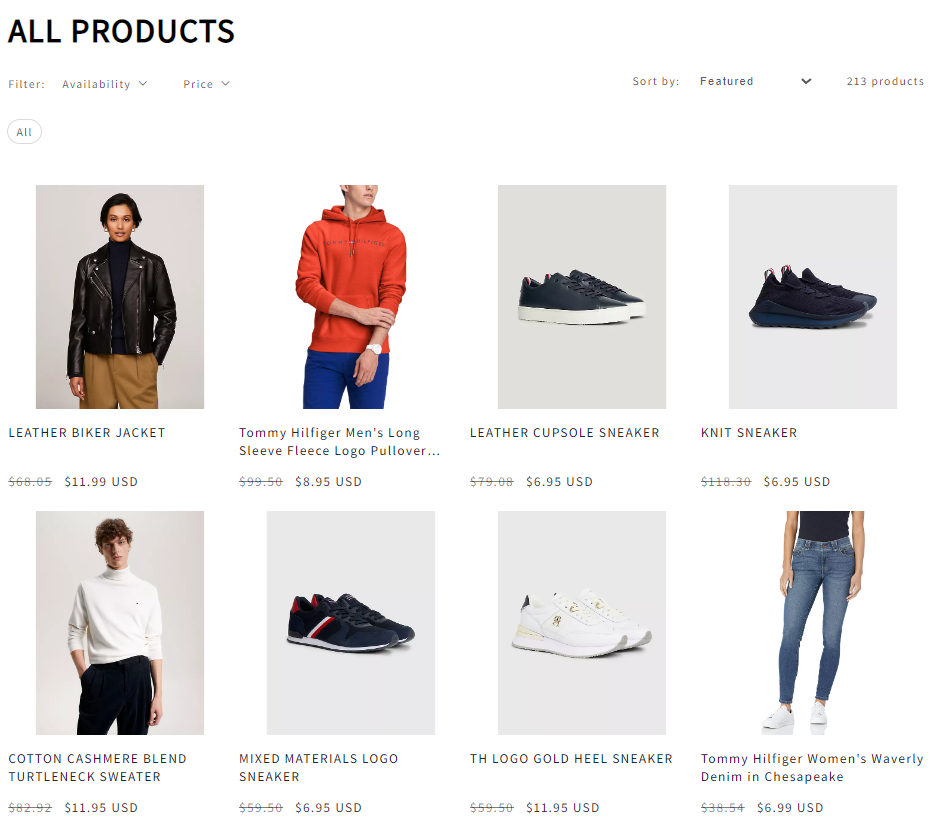This image is a screenshot from an online clothing and shoe retail website. The background of the webpage is white, and at the top in black text, it reads "All Products." Directly beneath this are options for "Filter," "Availability," and "Price" for easier navigation. Below these options is a blank space, followed by another row with "Sort By" and the default selection of "Featured." This line also indicates that there are 213 products available.

Displayed within the main section of the page are eight product images arranged in a 2x4 grid. In the top row, the first product is a "Leather Biker Jacket" modeled by a woman with her hand in her pocket. The second image is of a "Tommy Hilfiger Men's Long Sleeve Fleece Logo Pullover," which is a reddish-orange hue, worn by a male model. The third product is a "Leather Cup Sole Sneaker," characterized by its black upper and white sole. The fourth image in this row features a "Knit Sneaker," entirely black, including the sole.

The second row starts with a "Cotton Cashmere Blend Turtleneck Sweater." Next is a "Mixed Materials Logo Sneaker." The third image showcases a "Logo Gold Heel Sneaker." Finally, the last product in the row is "Tommy Hilfiger Women's Waverly Denim in Chesapeake." Each product is accompanied by high-quality images highlighting their key features for potential buyers.